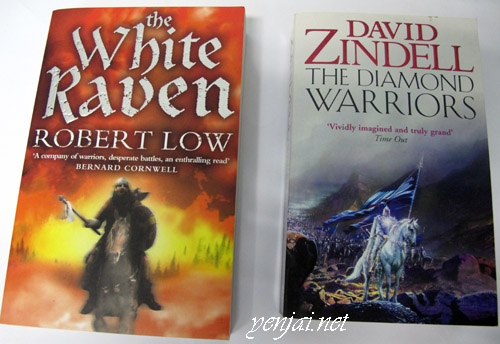In this photograph, two book covers are positioned side-by-side on a white background. The book on the left, titled "The White Raven" by Robert Lowe, features an intense fiery scene in shades of orange and yellow, resembling flames. The stark white title contrasts vividly with the blazing backdrop. Below the title and author's name, the cover depicts a figure riding a white horse, clad in dark attire with white headgear. The figure, possibly resembling a Viking, is holding what appears to be a spear or weapon. The entire scene is enveloped in a fiery ambiance.

The book on the right, titled "The Diamond Warriors" by David Zindel, has a predominantly white cover with the title in black and the author's name in large red letters at the top. The cover illustration showcases a white-clad figure riding a white horse, holding a blue banner. The backdrop features a gray and blue mountainous landscape, with rocky terrain under the horse's hooves. At the bottom of the cover, there is a mention of a website, benji.net, in small print.